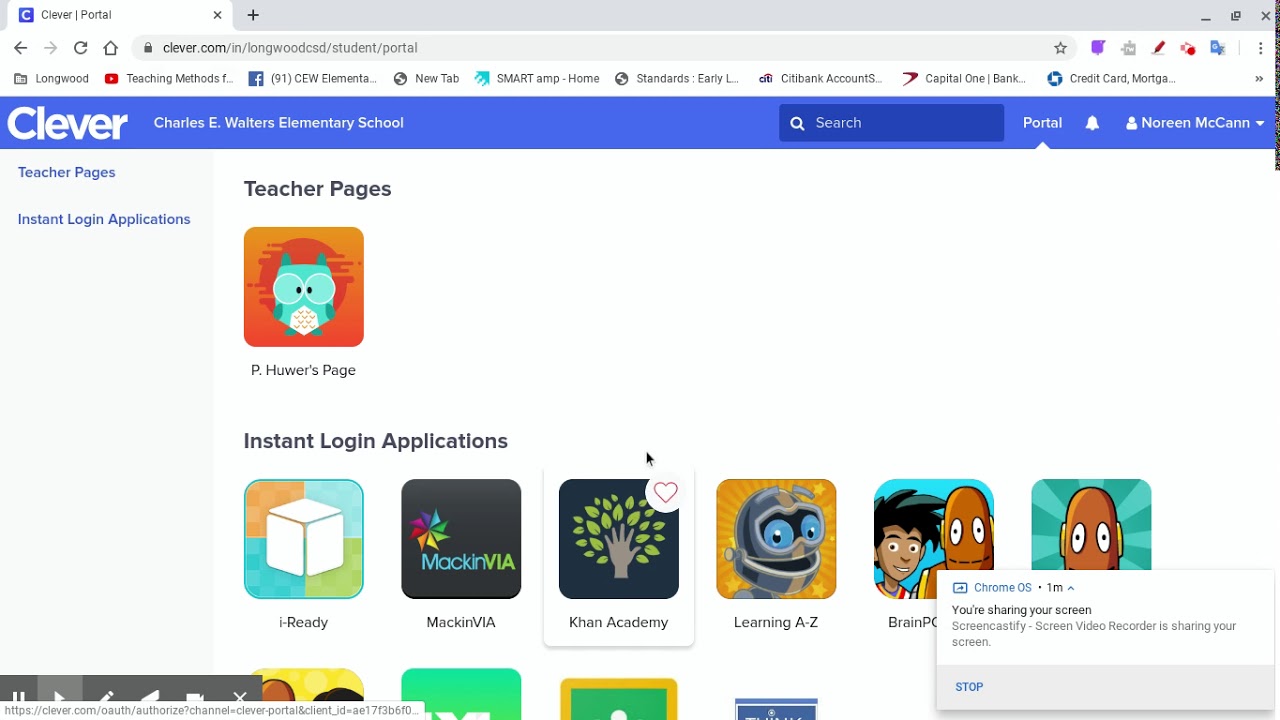This is a detailed screenshot of the Charles E. Walters Elementary School's Clever student portal homepage. At the very top, the browser tab reads "Clever / Portal" accompanied by a blue icon featuring a white "C" inside. The header section contains the options to search and access the portal, along with the user's name, "Noreen McCann," next to a drop-down menu icon.

On the left side, heading sections titled "Teacher Pages" and "Instant Login Applications" are prominently displayed. The first entry under "Teacher Pages" is an icon labeled "P. Hewer's Page," illustrated with a green cartoon owl set against an orange sun.

Below, the "Instant Login Applications" section features a row of six application icons. The first icon depicts a cardboard box, the second is labeled "MackinVIA" with a rainbow-colored design, the third is "Khan Academy" showcasing a hand and tree leaves, the fourth icon represents "Learning A-Z" with a robot image, the fifth reads "BrainPOP" (misstated as "Brain PC" in the original description), and the sixth partially hidden icon due to the screen-sharing overlay button does not have its software name mentioned.

Overall, the screenshot effectively showcases the organized layout of education resource links provided through the school’s Clever portal, designed to facilitate student access to their personalized educational tools and teacher pages.